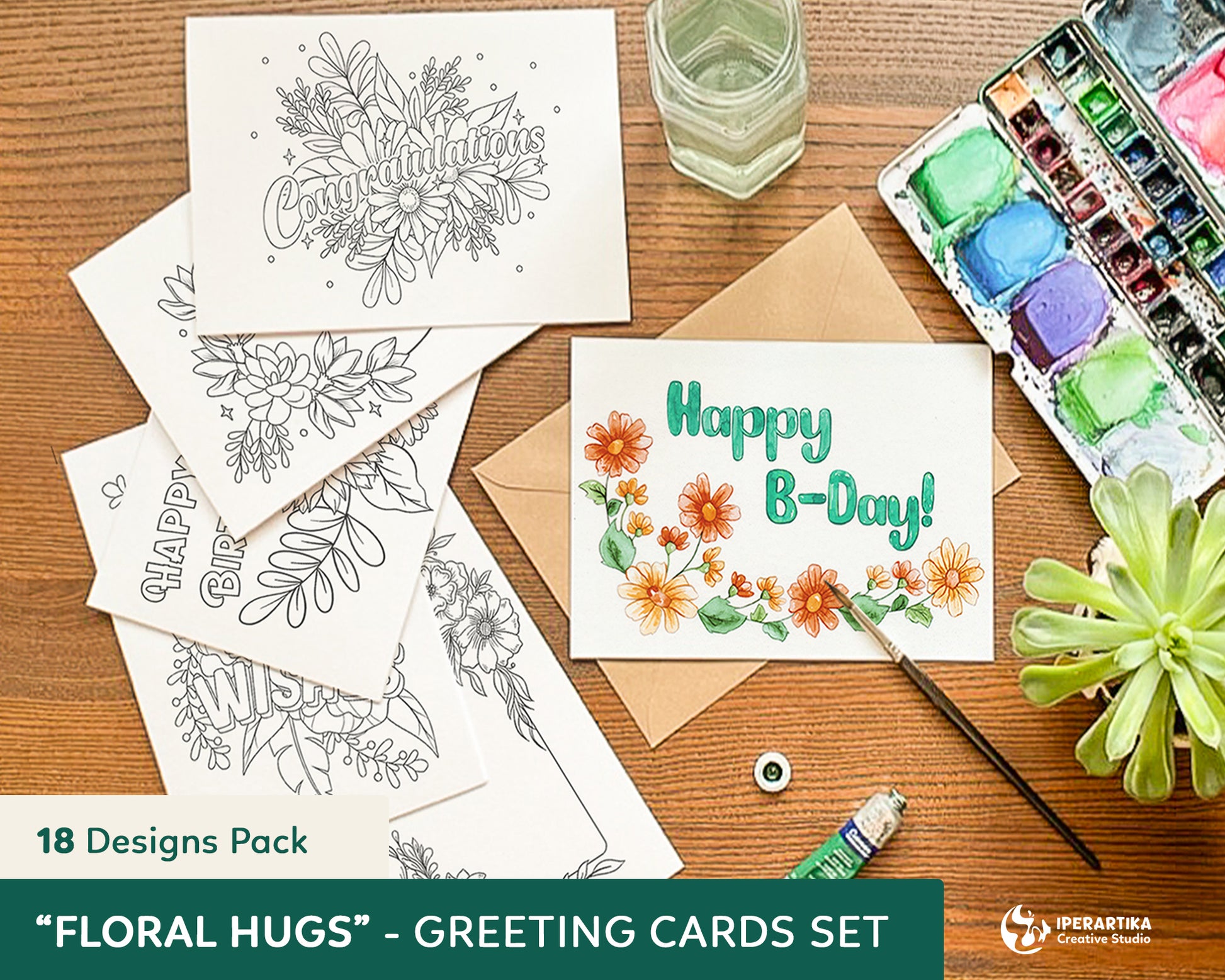This large, square image showcases a medium brown desk with darker horizontal grains. At the top center, a glass jar partially filled with water sits, likely used for rinsing paintbrushes. To the upper right, a palette of messy, used watercolors featuring various hues such as green, purple, and blue hints at recent creative activity. The focal point in the center is a white envelope featuring a hand-painted "Happy B-day!" in green, adorned with a string of roses transitioning from red to orange to yellow. This envelope has a paintbrush resting on top. Below it, there’s an open tube of paint. Scattered across the desk, overlapping papers reveal black-and-white floral designs waiting to be colored, with messages such as "Congratulations," "Happy Birthday," and "Best Wishes." In the lower-left corner of the image, text reads "18 Designs Pack" in green against a white background, and "Floral Hugs – Greeting Card Set" in white against a green background. The presence of a small succulent plant adds a touch of nature to the artistic workspace.